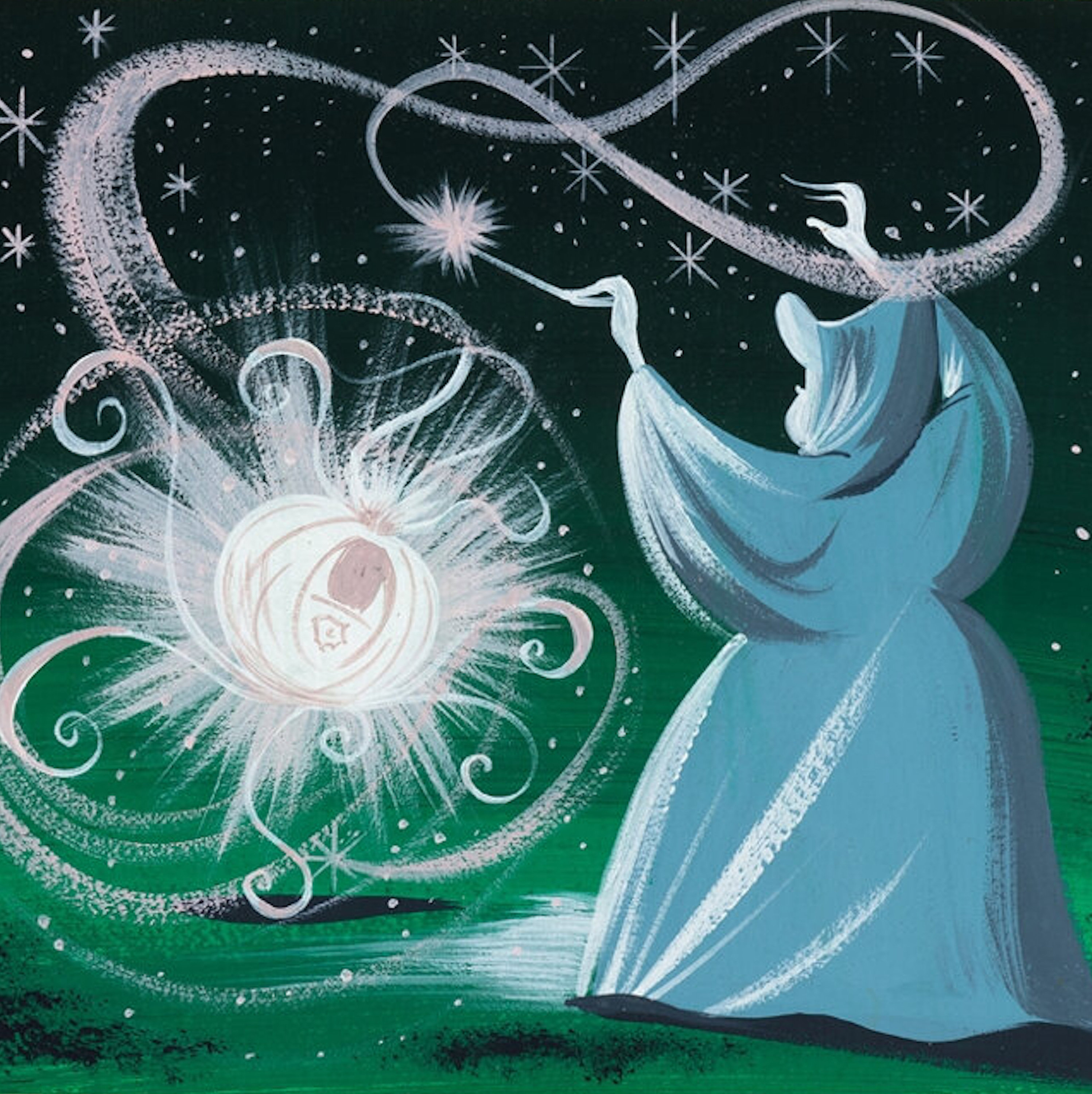This image depicts an enchanting scene from the Cinderella fairy tale, illustrating the Fairy Godmother in the act of transforming a pumpkin into a carriage. Set against a deep green, almost black night sky dotted with simple, white crayon-textured stars, the scene exudes a magical atmosphere. The Fairy Godmother herself, cloaked in a heavy, billowing robe of turquoise and seafoam blue with a hood obscuring her face, holds a white wand aloft in her left hand. Swirls of sparkling light emanate from the wand, sweeping across the upper part of the image before descending to the left, converging into the preliminary form of a pumpkin, signifying the transformative magic at work. The ground beneath features a textured green, suggestive of grass, which contrasts with the dark background, emphasizing the magical light trails that dominate the scene.